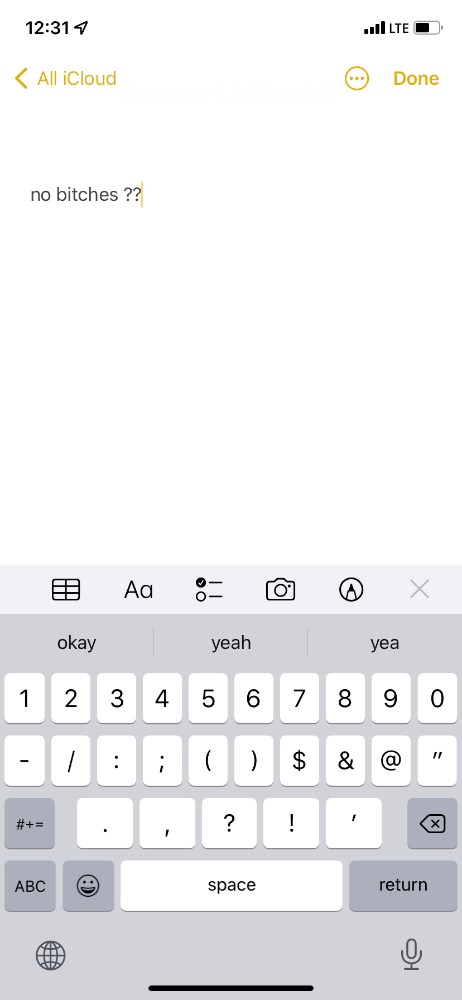The image depicts a close-up of a smartphone screen. The status bar at the top indicates the device is operating on an LTE network with full signal strength, and the battery level is at 50%. The time displayed is 12:31 PM. Beneath the time, there is a line of text in yellow that reads "All Cloud." 

On the left side of the status bar, there is a back arrow symbol, and on the right, there is a "Done" button also highlighted in gold. Just below these elements, a circular icon with three vertical dots is visible. 

The main area of the screen shows the text "No bitches??" followed by a small vertical line in gold. Directly below this message, a keyboard is present. The keyboard suggests three words: "okay," "yeah," and "yea." At the top edge of the keyboard, there are several icons, including a capital 'A' inside a circle, an 'X,' a camera, two dots connected by lines, a larger capital 'A,' a smaller lowercase 'a,' and a box with lines inside it.

The keyboard itself appears to be a traditional QWERTY layout, featuring numbers, special characters like the dollar sign and at symbol (@), as well as space and return keys at the bottom. Additional functionality is provided by icons for voice input (microphone) and internet access (World Wide Web symbol).